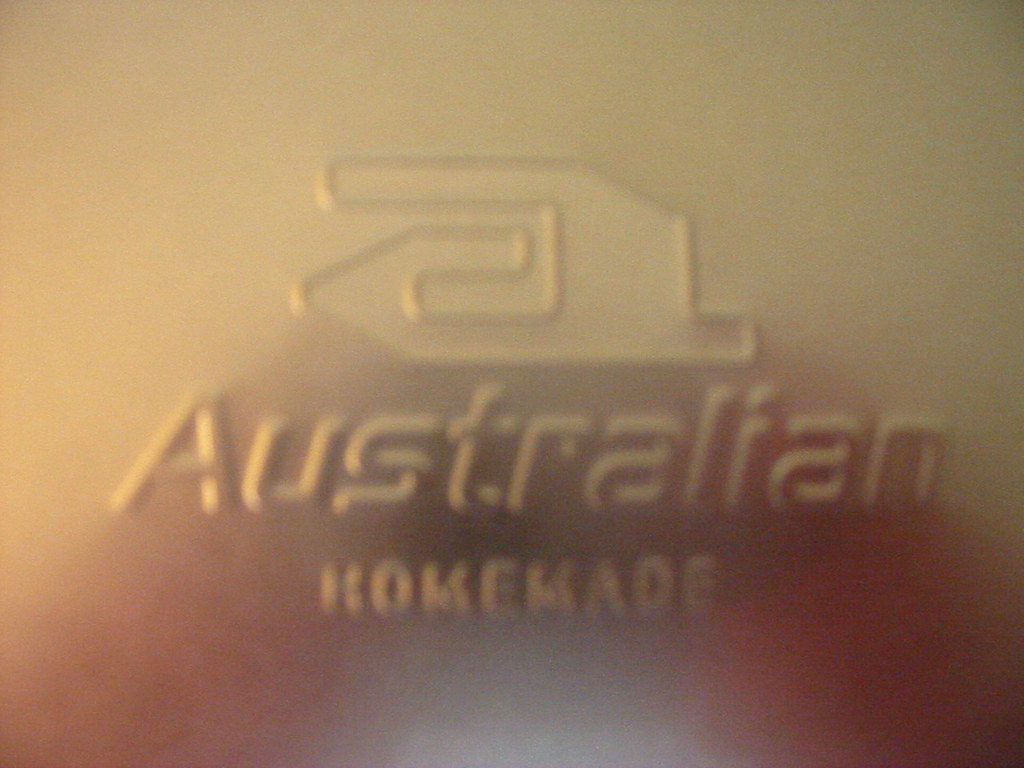This photograph captures an embossed metal logo, which features a prominent lowercase "a" as its main design element. Below the "a," the word "Australian" is inscribed in a more conventional font. Further down, in much smaller and uppercase letters, the phrase "HOME MADE" appears. The logo stands out against the silver-colored metal surface, which has been embossed from the back to create a raised effect. The image is notably blurry and lacks focus, making the details hard to discern clearly. The metal reflects various colors, including brown and a mustard yellow hue, likely due to surrounding ambient lighting. A faint reflection of the person who took the photograph can be seen at the bottom of the image.